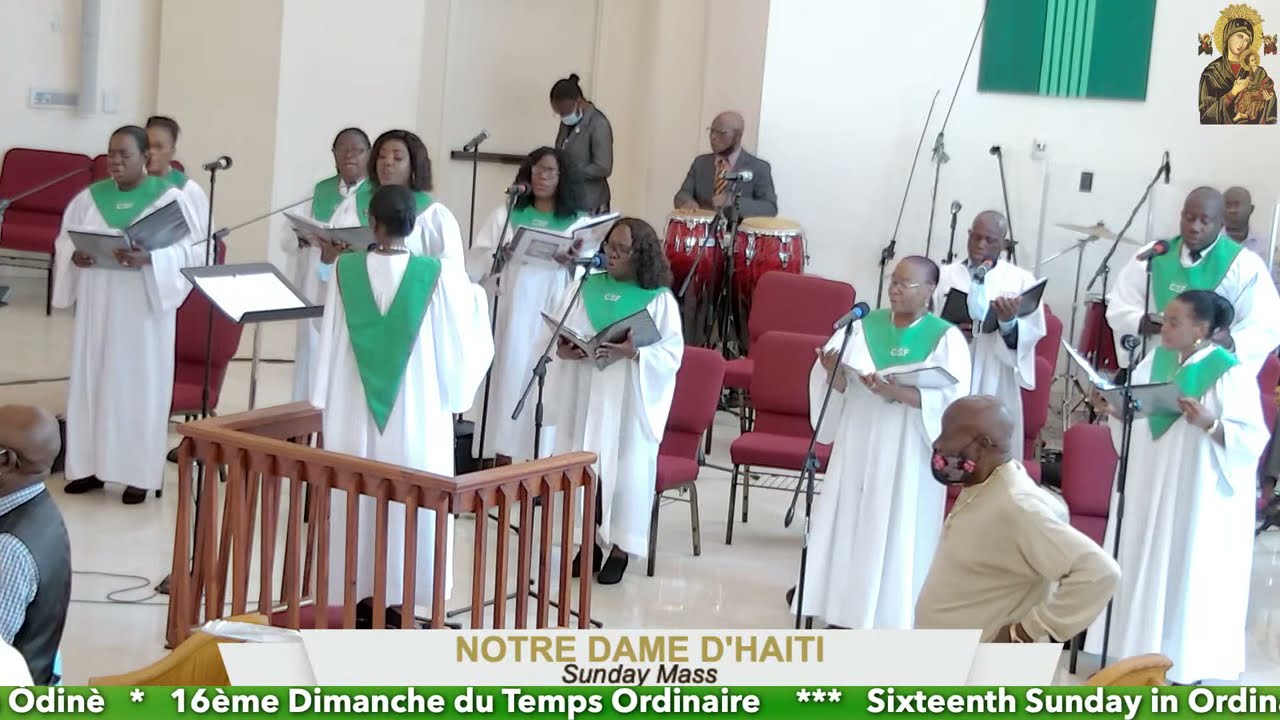The image depicts a television broadcast still frame of a Haitian choir performing during the Notre Dame de Haiti Sunday Mass, identified as the 16th Sunday in Ordinary Time. The choir, composed of approximately ten to twelve members, predominantly women with only a few men, is dressed in white robes adorned with green stoles that drape in a V-shape down their chests. Each member holds a binder or hymnal from which they are singing. In the foreground, the choir director stands facing the choir, presumably conducting them. Behind the choir, a small band is visible, including a man playing conga drums and another seated at a drum set. Notably, one man in the scene is wearing a face mask. The bottom of the image features a white caption with gold lettering that reads "Notre Dame de Haiti Sunday Mass" with a French translation "16ème Dimanche du Temps Ordinaire" indicating the specific mass being celebrated.